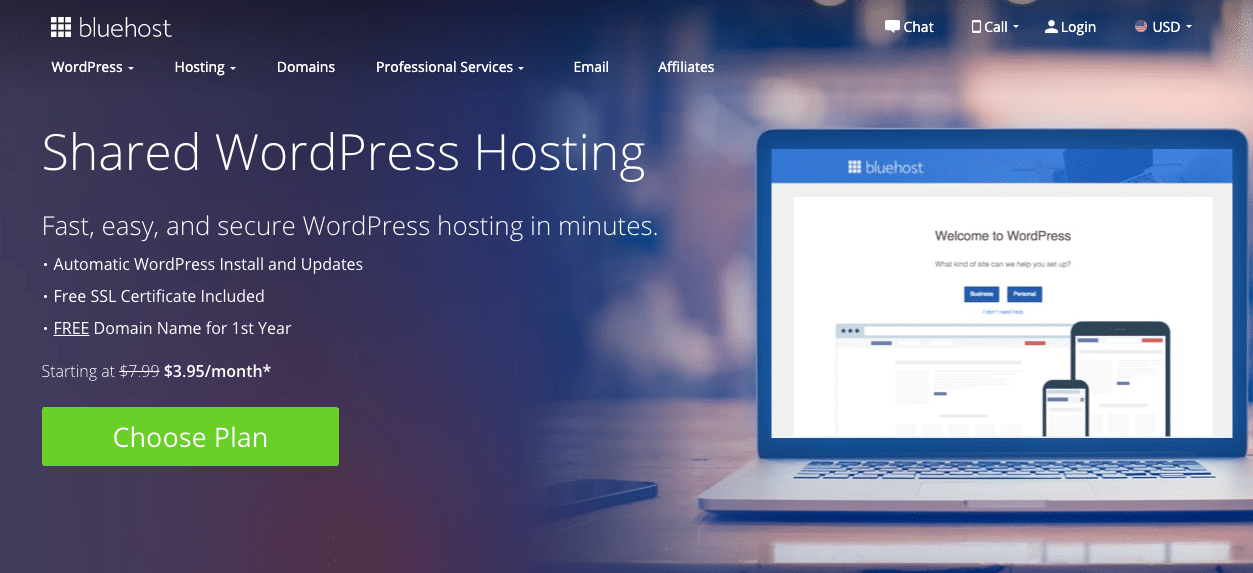Screenshot of the Bluehost website:

At the top left, the Bluehost logo is displayed in white alongside an icon consisting of a grid with nine small white squares. Beneath the logo, the navigation menu includes the following options: "WordPress," "Hosting," "Domains," "Professional Services," "Email," and "Affiliates."

The main header section prominently features the text "Shared WordPress Hosting" in large font. Directly below, smaller text describes the service as "fast, easy, and secure WordPress hosting in minutes."

A bullet-point list highlights the following features:
- Automatic WordPress install and updates.
- Free SSL certificate included.
- Free domain name for the first year.

The original price of $7.99 per month is crossed out and replaced with a sale price of $3.95 per month, marked with an asterisk. Below this pricing information, there is a green rectangular button with white text that reads "Choose Plan."

To the right of the textual content, an image of a laptop is displayed, complementing the website’s technological theme.